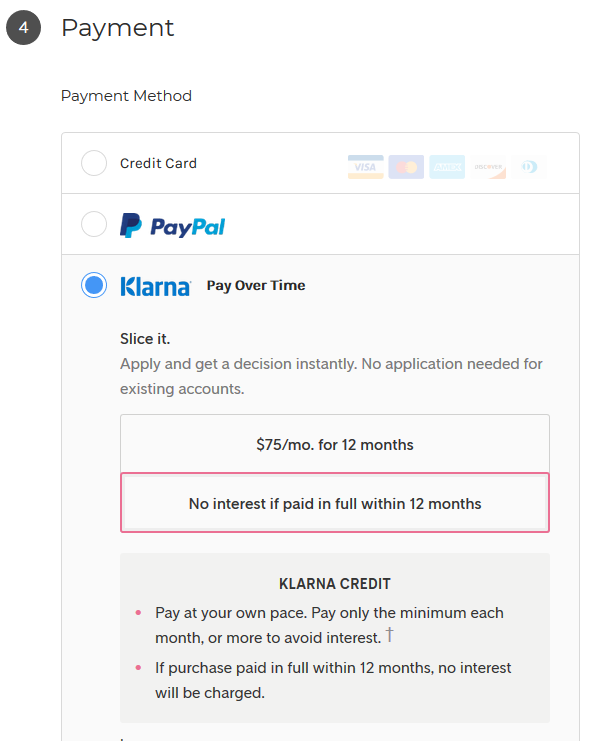In this detailed screenshot image of a purchase screen, the upper left corner features a grey circle with a white number "4" inside it, indicating the fourth step in the purchase process. To the right of this circle, the word "Payment" is prominently displayed. Beneath this heading, the section is labeled "Payment Method," showcasing various payment options available for selection.

At the top of the payment options list is "Credit Card," accompanied by icons representing Visa, MasterCard, American Express (Amex), and Discover cards. Following this is another payment option marked by a blue circle with white letters inside. The next option listed is the PayPal logo, easily recognizable for users who prefer this payment method.

The final payment option provided, which is selected in this screenshot, is Klarna. This option has the tagline "Pay Over Time. Slice It," emphasizing flexible payment plans. Detailed instructions underneath explain that users can "Apply and get a decision instantly," with no application needed for existing accounts. Klarna offers two primary payment plans: "$75 a month for 12 months" or "No interest if paid within 12 months," the latter of which is highlighted within a red rectangle for emphasis.

Additionally, the section elaborates on Klarna Credit, stating "Pay at your own pace. Pay only the minimum each month or more to avoid interest. If the purchase is paid in full within 12 months, no interest will be charged," providing clear terms to the user.

The structured and comprehensive format of the information ensures that buyers can easily understand and choose their preferred payment method.